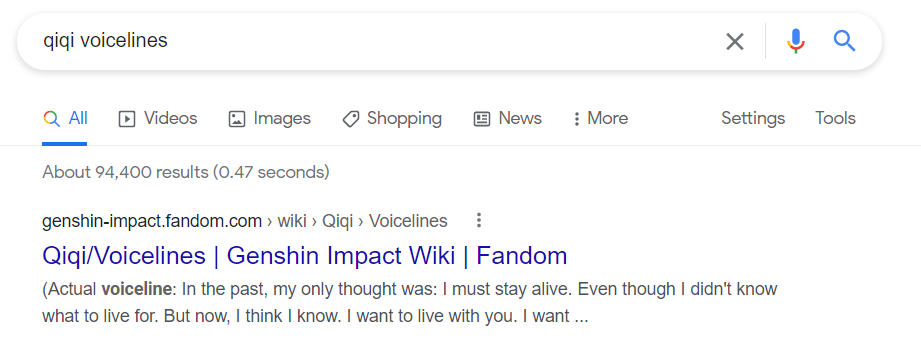The image showcases a Google search interface on a white background. At the top of the image is the search bar, featuring a grey "X" icon to clear the search box, and a colorful microphone icon in blue, yellow, red, and green, allowing for voice search. Situated beside these icons is a blue search button. Within the search bar, the user has typed "Qiqi voice lines." This text is displayed in black font.

Underneath the search bar, a series of tabs is present: "All," "Videos," "Images," "Shopping," "News," "More," "Settings," and "Tools." The "All" tab is in blue to indicate it is currently selected, while the other tabs are in grey. Below these tabs, the search indicates there are approximately 94,100 results, retrieved in 0.47 seconds.

The first result is a link to the Genshin Impact wiki on Fandom. The URL, "GenshinImpact.Fandom.com/wiki/Qiqi_voice_lines," is displayed underneath the title in green text. The clickable heading "Qiqi/Voice Lines - Genshin Impact Wiki - Fandom" is written in blue with a slight purple tint, suggesting that it has been previously visited. The snippet from the webpage reads, "Actual voice line: In the past, my only thought was I must stay alive, even though I didn't know what to live for. But now, I think I know. I want to live with you."